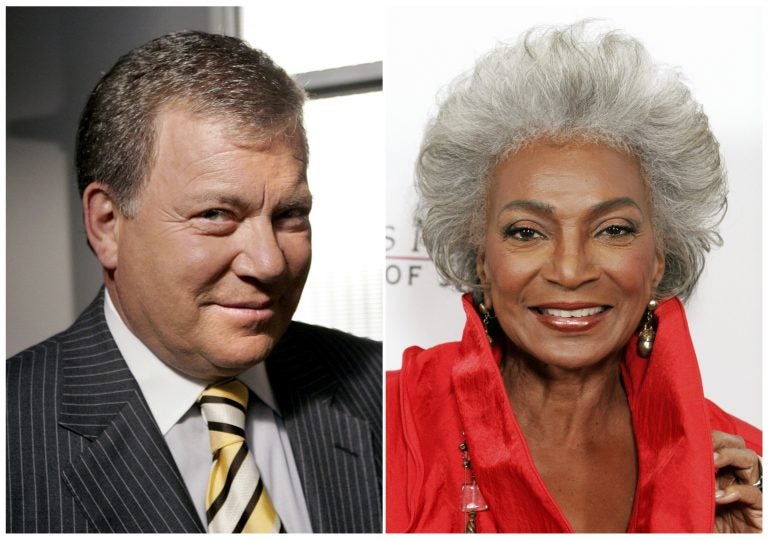This image showcases two famous actors side-by-side. On the left, we have William Shatner, known for his role as Denny Crane in the TV show Boston Legal, among other roles. Shatner has graying dark hair and is wearing a black suit with white pinstripes, paired with a white button-up shirt and a distinctive tie featuring black, yellow, and white stripes. He is smiling directly at the camera, giving a somewhat sinister yet charming look. The background behind him features a gray wall with a window on the right side, framed in light gray, which adds depth to the lighting.

On the right side of the image, we see an African American woman portrayed by the actress who played the communications officer, Uhura, in the original Star Trek series. She has mocha-toned skin and a fluffy, poofy hairstyle that is predominantly gray with white streaks. She is wearing a vibrant red high-collared outfit, possibly a dress or jacket, which complements her shiny lips and dark eyebrows. Her accessories include dangling gold earrings, a gold necklace, and a silver ring on her marriage finger. The background behind her is predominantly white, featuring some black text and a red light that suggests she might be at a notable event, possibly a film festival. She is smiling warmly, directly facing the camera.